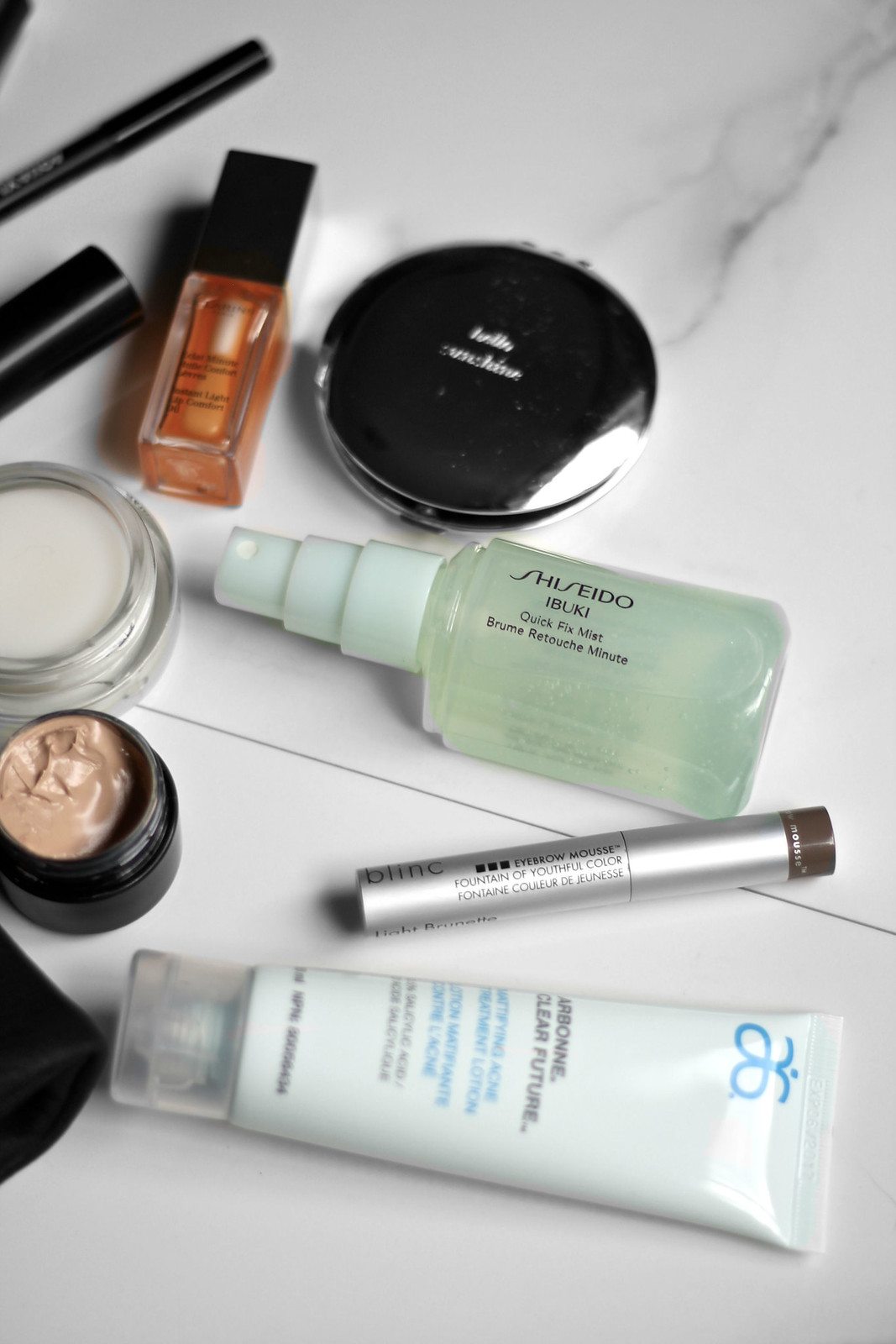On a pristine white marble countertop adorned with dark veining, several cosmetics are artfully arranged. The marble surface is divided by a distinctive black line running horizontally across the middle, indicating the joining of two stone pieces. In the vertical-format image, the top left corner reveals a small smidge of black, hinting at another cosmetic item just out of frame. Emerging diagonally from the upper part of the scene is part of a black eye pencil. Below it appears a partially visible black tube, which could either be a lipstick or the top of a mascara. Centrally positioned is a square bottle filled with amber fluid, standing next to a sleek black compact. A shiny silver container holds face cream, and placed horizontally is a mint-green spray bottle labeled "Shishito." Additionally, a silver eye pencil, a small white tube of cream, and a black foundation container occupy the left side of the composition.